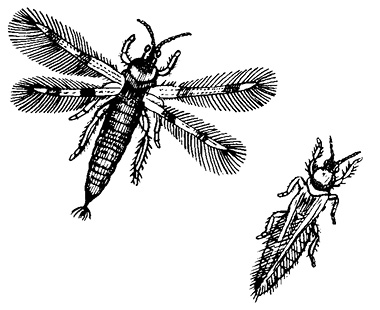This black-and-white illustration showcases two detailed forms of an insect set against a stark white background. In the upper left of the image, the insect is depicted ready to take flight, with its four delicately detailed wings spread out, resembling feathers. This form highlights the insect’s long, segmented abdomen adorned with fine lines, its thick antennae, prominent eyes, tiny head, hairy legs, and open mouth. In the bottom right, the same insect is illustrated with its wings folded back, accentuating the sleek and elongated silhouette of its body. Both renditions are meticulously drawn, capturing intricate details like the six legs and segmented wings.